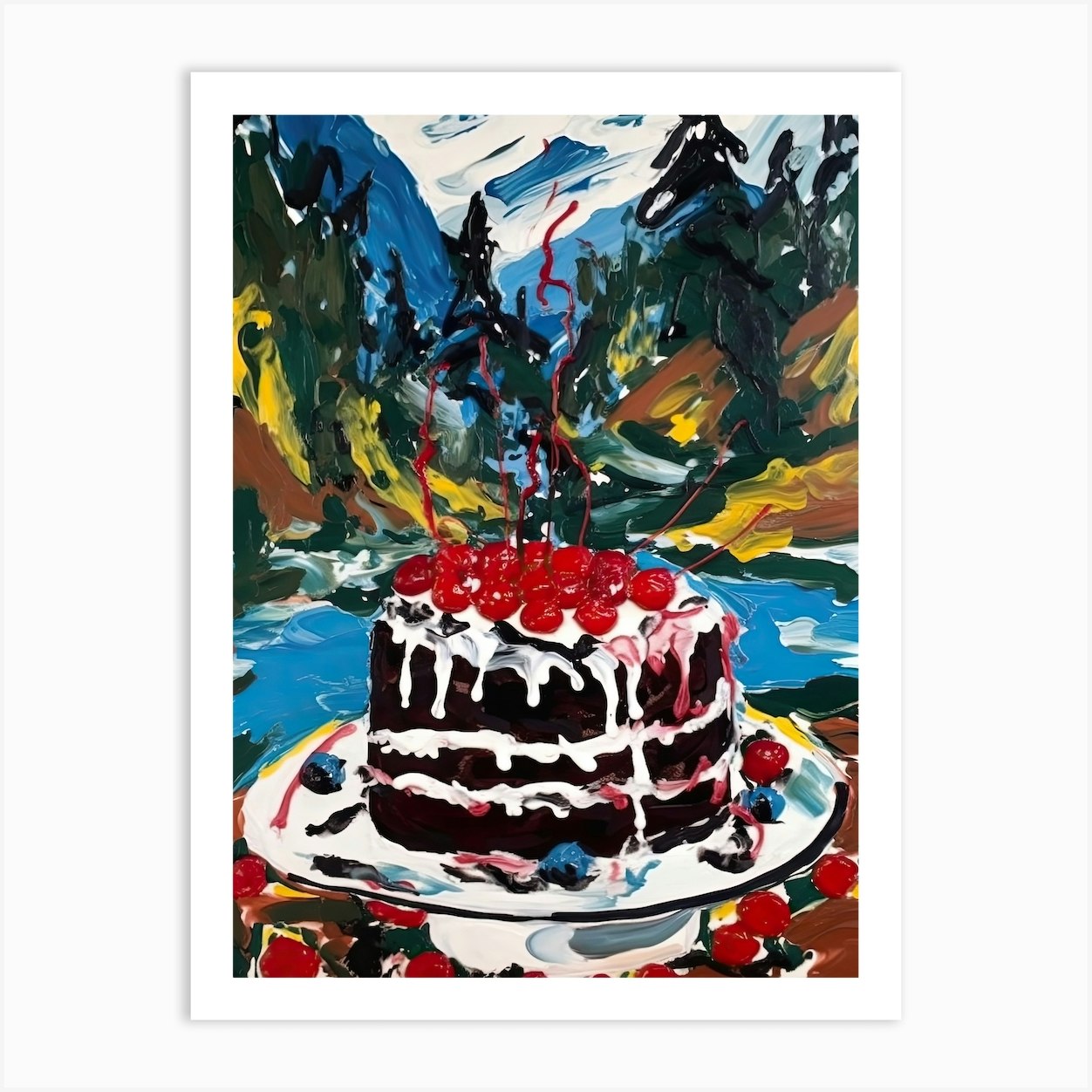The painting, elegantly encased in a pristine white frame, depicts a sumptuous chocolate cake adorned with luscious white layers, likely frosting or whipped cream, that drip down its sides. Topping the cake are vibrant maraschino cherries, some of which have tumbled off the white cake stand with a black rim onto the foreground. The backdrop of the artwork is a vivid and dynamic landscape with a body of blue water, white and blue mountains, and a mix of brown, yellow, and green hues suggesting trees and natural scenery. The scene combines the indulgence of the dessert with the serenity of the natural elements, adding a rich context to this delectable portrayal.